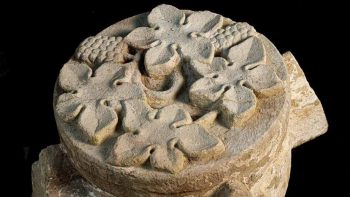This photograph showcases an ancient archaeological artifact—a roundel sculpted from a light-colored stone. The roundel features a detailed relief carving of grape leaves arranged in a radiating pattern, interspersed with plump, realistic grape clusters. The stone's surface displays spots of a darker hue, adding depth to the piece. The carving is three-dimensional and intricately detailed, suggesting the craftsmanship of a highly skilled artisan. Surrounding the roundel, a horizontal shape juts out from the lower left to the upper right, adding to the artifact's complexity. The artifact is professionally photographed against a black background, highlighting every nuance of its design. This piece, reminiscent of artwork found in prestigious galleries or museums, exudes an aura of antiquity, likely dating back hundreds or even thousands of years. The absence of contextual text leaves its exact origins and purpose open to interpretation.